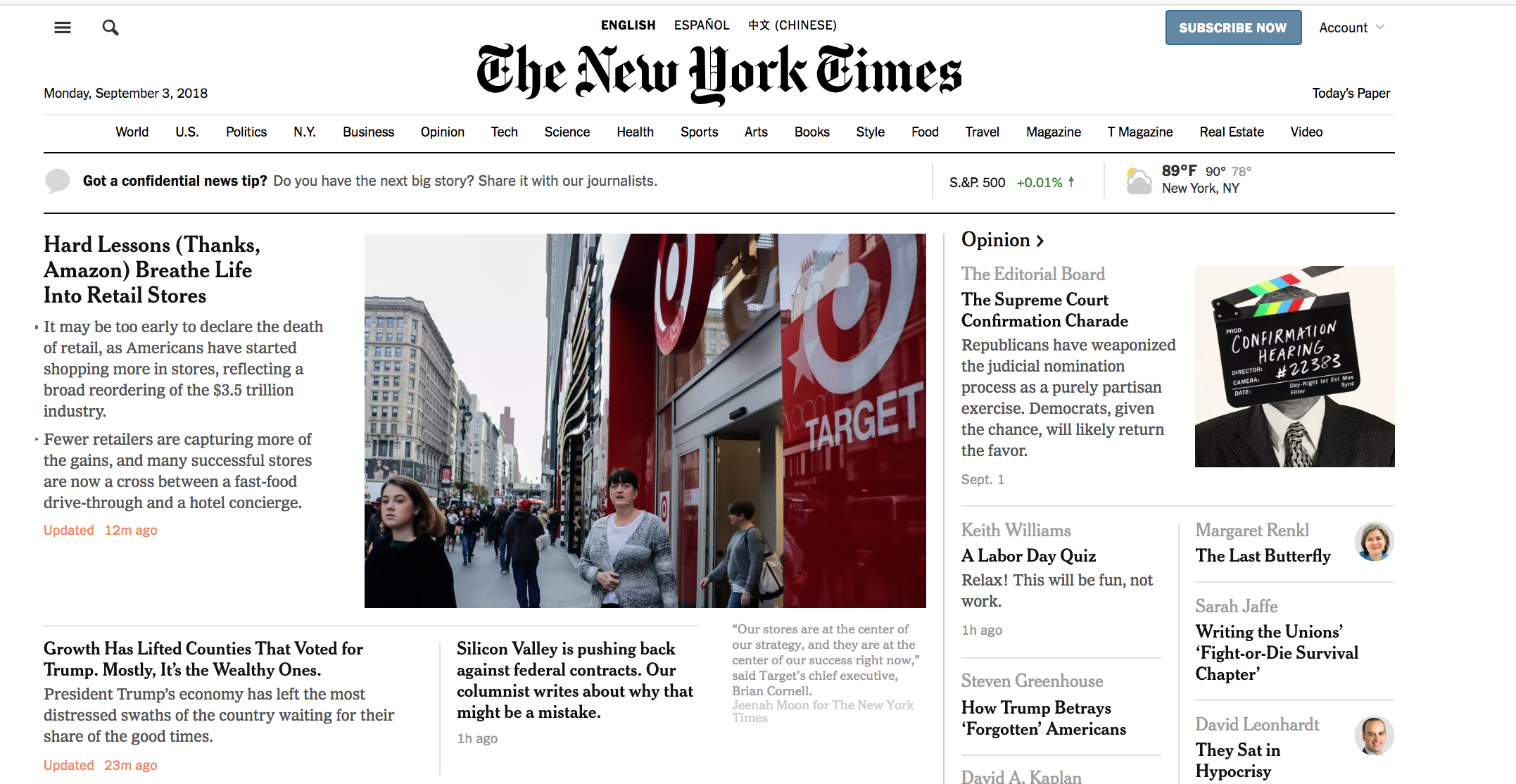The webpage of the New York Times features a detailed layout starting with three horizontal dots, a magnifying glass icon, and a language selection for English, Español, and Chinese. A blue "Subscribe Now" button is prominently displayed, followed by an "Account" drop-down menu. The date, Monday, September 3rd, 2018, is presented on the next line alongside 'The New York Times' title in a stylized font and a link to "Today's Paper". Beneath this is a section inviting confidential news tips and S&P numbers, along with weather information specific to New York, New York.

Centrally placed on the page is an image depicting a downtown street in New York, dominated by several retail stores, most notably Target. Below the image, prominent headlines include "Hard Lessons: Thanks Amazon, Breathe Life Into Retail Stores" and "Growth Has Lifted Countries That Voted For Trump, Mostly It's The Wealthy Ones." Another key headline reads "Silicon Valley Is Pushing Back Against Federal Contracts, Our Columnist Writes About Why That Might Be A Mistake." The opinion section features headlines such as "A Labor Day Quiz: How Trump Betrays Forgotten Americans," "The Last Butterfly," "Writing the Union's Fight or Die Survival Chapter," and a critique stating "They Sat in Hypocrisy."